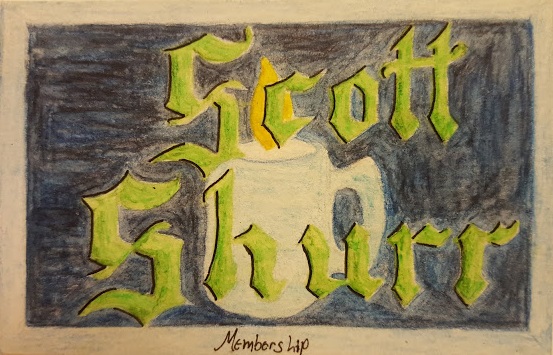The image depicts a drawing on tan-colored paper, created using either pencil crayons or wax crayons. Dominating the composition is a black, filled-in rectangle positioned at the center of the sheet. Within this rectangle, a white candle, designed to resemble a coffee mug, stands prominently, its flame flickering towards the top. Encircling the candle, in eerie green letters with a black outline, are the words "Scott Schur." Beneath the black rectangle, directly on the tan area of the paper, the word "membership" is inscribed in black writing. The overall color scheme is a striking combination of black, tan, and green, creating a haunting yet intriguing visual contrast.